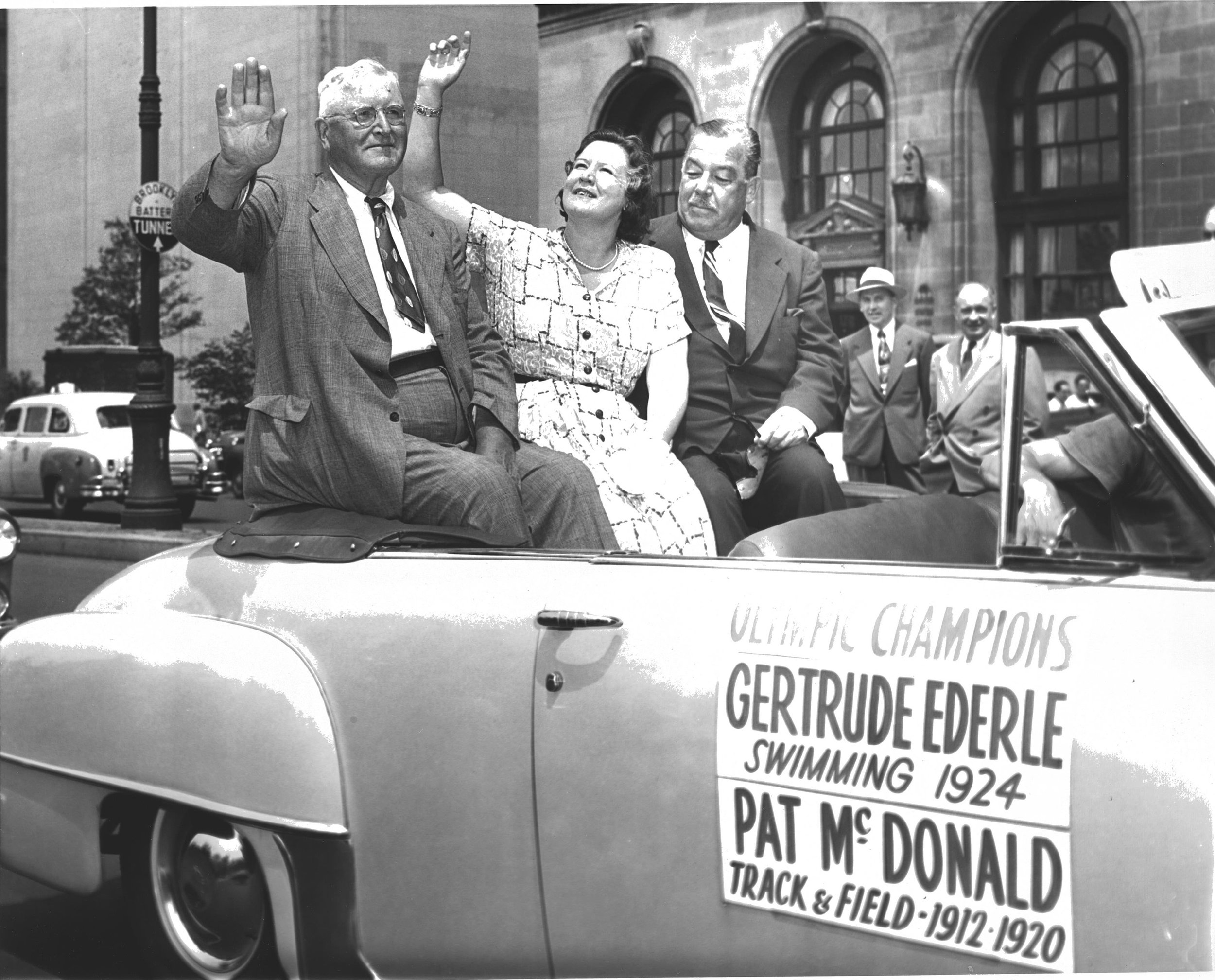This detailed black and white photograph appears to be from the 1950s and captures a lively moment during a parade. Sitting atop the back of a convertible vehicle, three celebrated individuals are prominently featured: two older gentlemen and a woman seated between them, identified by the sign on the side of the car as Olympic champions Gertrude Ederle, renowned for swimming in 1924, and Pat McDonald, distinguished in track and field from 1912 to 1920. The gentleman on the far left, sporting white hair, glasses, and a polka dot tie, is joyfully waving with his right arm outstretched, his closed-mouth smile endorsing the jubilant atmosphere. Similarly, the elegantly dressed woman in the middle, wearing a white tweed dress with black squares and a simple necklace, raises her right hand to wave at the onlookers. The second gentleman on the right, who holds sunglasses in his lap, is directed toward the woman, creating a sense of connection among the trio. Behind them, an older masonry stone building with imposing arched windows and a giant doorway, an old streetlight pole, and a classic taxi set the nostalgic scene. On the sidewalk, several men in suits observe the event, their attention captured by the procession. The right arm and elbow of the convertible's driver are faintly visible on the image's far right, adding depth to this captivating snapshot of history.